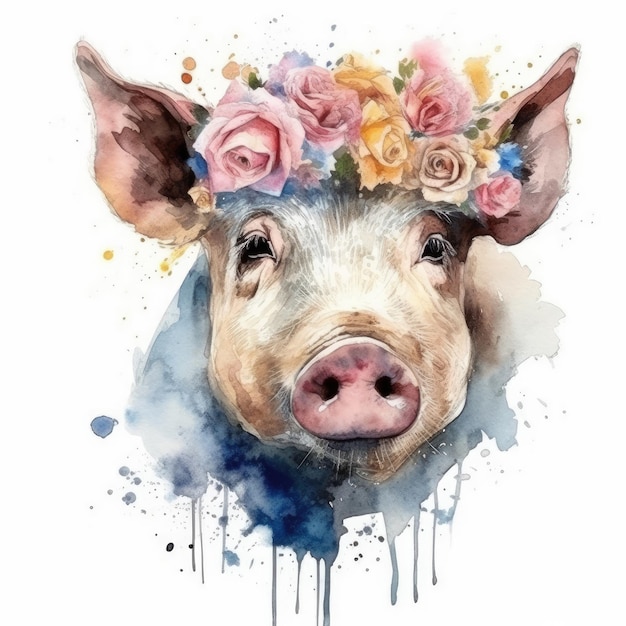This detailed watercolor image showcases the face of a pig adorned with a vibrant crown of roses in hues of pink, salmon, purple, blue, and hints of yellow. The pig's expressive eyes, visible eyelashes, and delightfully large ears lifted as though savoring a pleasant sound, convey a serene and content demeanor. The artistic rendering captures fine details such as the crevices of the pig's big pink nose and delicate whiskers, emphasizing the artist's skill. The pig's predominantly pink complexion includes patches of white around its snout, further adding to its charm. Surrounding the pig's head, the background features blue splotches and splashes of roses’ colors, with watercolor paint artfully dripping down from the chin, accentuating the medium's fluid nature. The overall composition presents a beautifully detailed pig face, staring directly at the viewer, exuding a peaceful and joyful essence.